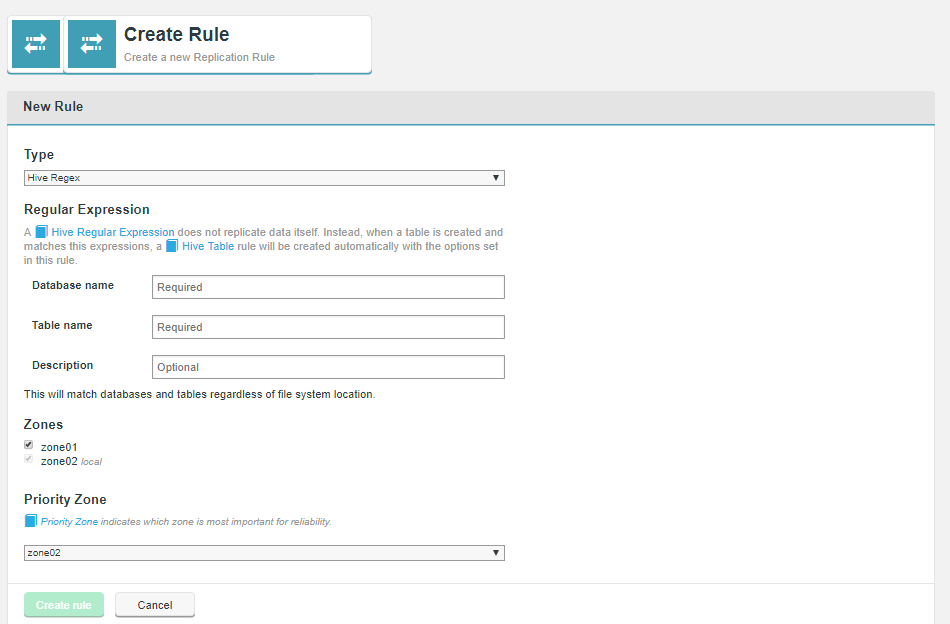The image displays a webpage, clearly a part of a site dedicated to creating rules for replication. Prominently at the top, two aqua blue boxes feature arrows; the upper arrow points to the right and the lower arrow points to the left, each with decorative lines on their tails. Adjacent to these boxes, bold black text reads "Create Rule," followed by the subtext "Create a new replication rule" within a long, white rectangular box.

Beneath this, the layout transitions into a grayed-out section, leading to a darker gray area labeled "New Rule." Here, the term "Type" appears above a lengthy drop-down box displaying the option "Hive REGEX" (Regex likely spelled as R-E-G-E-X). Following this, a paragraph containing highlighted blue icons labeled "Hive regular expression" and "Hive table" provides an explanation. Further details prompt the user to enter information for "Database Name," "Table Name" (both marked as required), and "Description" (marked as optional) into designated input boxes.

The section labeled "Zones" shows a checkmark next to "Zone 01." At the bottom, the interface offers two buttons: "Create Rule" and "Cancel."